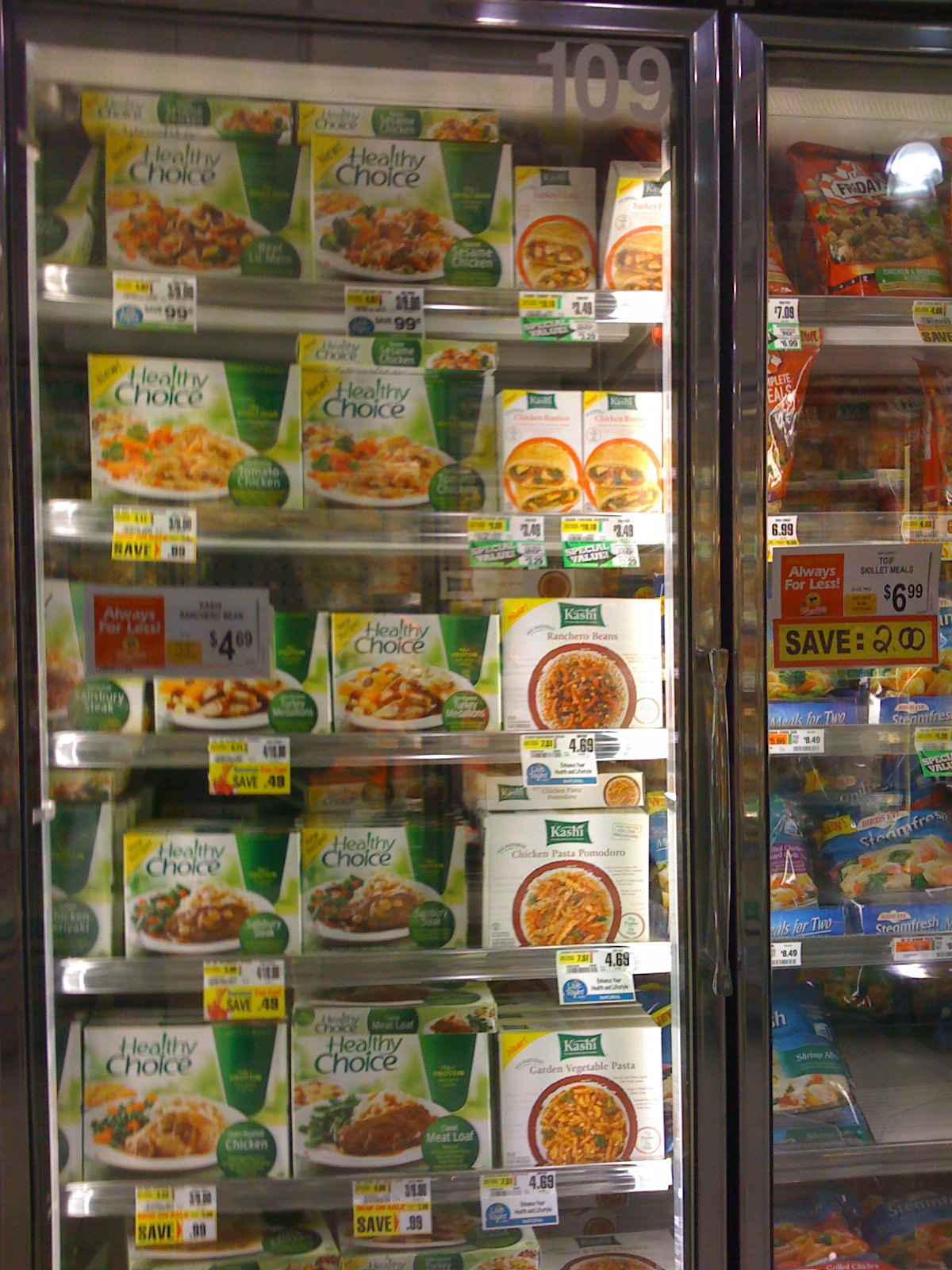A first-person point of view image taken within a grocery store showcases a close-up of the chilled and frozen food section through glass doors with distinctive red and black frames and black handles. The focal point is one prominent door, with about a quarter of an adjacent door visible on the right side. Above the main door, the number "109" is displayed in grey.

The shelves are stocked with a variety of frozen meals, primarily from the brand Healthy Choice. The top row features a sesame chicken flavor alongside a beef option. To the left of these, there's another sesame chicken meal. The second row holds tomato chicken meals, displayed twice. The first three rows highlight Healthy Choice products, each box adorned with a graphic of the meal and its flavor indicated in the bottom right corner.

On the right side of the display, a smaller, mostly unreadable white packet with a burger graphic appears next to some of the Healthy Choice options. This smaller packet continues in succession down the six rows of shelves, consistently occupying the right half while Healthy Choice meals dominate the left. The third row’s Healthy Choice offerings have labels that are too small to read, but the pattern of left-side Healthy Choice and right-side white packet persists through all six rows.